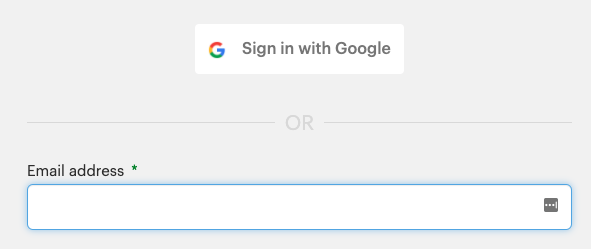The image is a small, minimalistic login interface set against a light gray background. At the very top center of the image is the multicolored "G" logo representing Google. Just below the logo is a white box with the text "Sign in with Google" in bold black letters, inviting users to log in using their Google account. Beneath this option, a thin line runs horizontally across the page. At the center of the line is the word "or" highlighting an alternative sign-in method. Directly below this, there is text indicating "Email address" followed by an asterisk, suggesting that this field is required. Adjacent to this text is an empty input field bordered by a highlighting blue line, where users can type in their email address. The image does not contain any additional information about the website or service for which the user is attempting to log in, maintaining a sparse and clean design with no further context or branding.